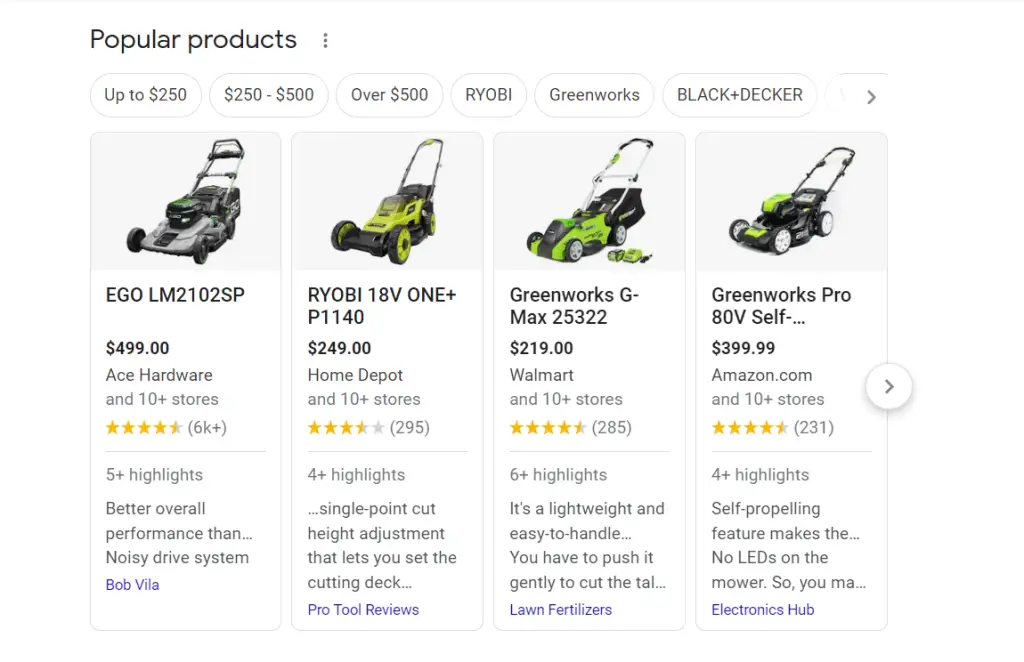This is a screenshot of a website displaying the "Popular Products" section, highlighted prominently at the top with three adjacent black dots. Directly beneath this heading are a series of filter bubbles containing black text on a white background, neatly aligned horizontally. The bubbles categorize the products by price and brand: the first bubble reads "Up to $250," the second "250 to $500," and the third "Over $500." Following the price filters, brand filters are listed as "RYOBI," "Greenworks," and "Black & Decker."

Below these filters are several shopping options for lawnmowers, each featuring a product image, price, retailer information, and star ratings. The first item is a gray-and-green lawnmower priced at $499, available from Ace Hardware. It displays star ratings underneath. To the right is another lawnmower, green and white, priced at $249 from Home Depot, following the same informative setup. Next, another green-and-white lawnmower is listed at $219 from Walmart, also showing its star ratings. The fourth option features a black-and-green Greenworks Pro lawnmower for $399.99, available from Amazon.com, complete with its rating system.

On the right-hand side of the page, there is an arrow within a bubble, seemingly a control to scroll for additional product options.